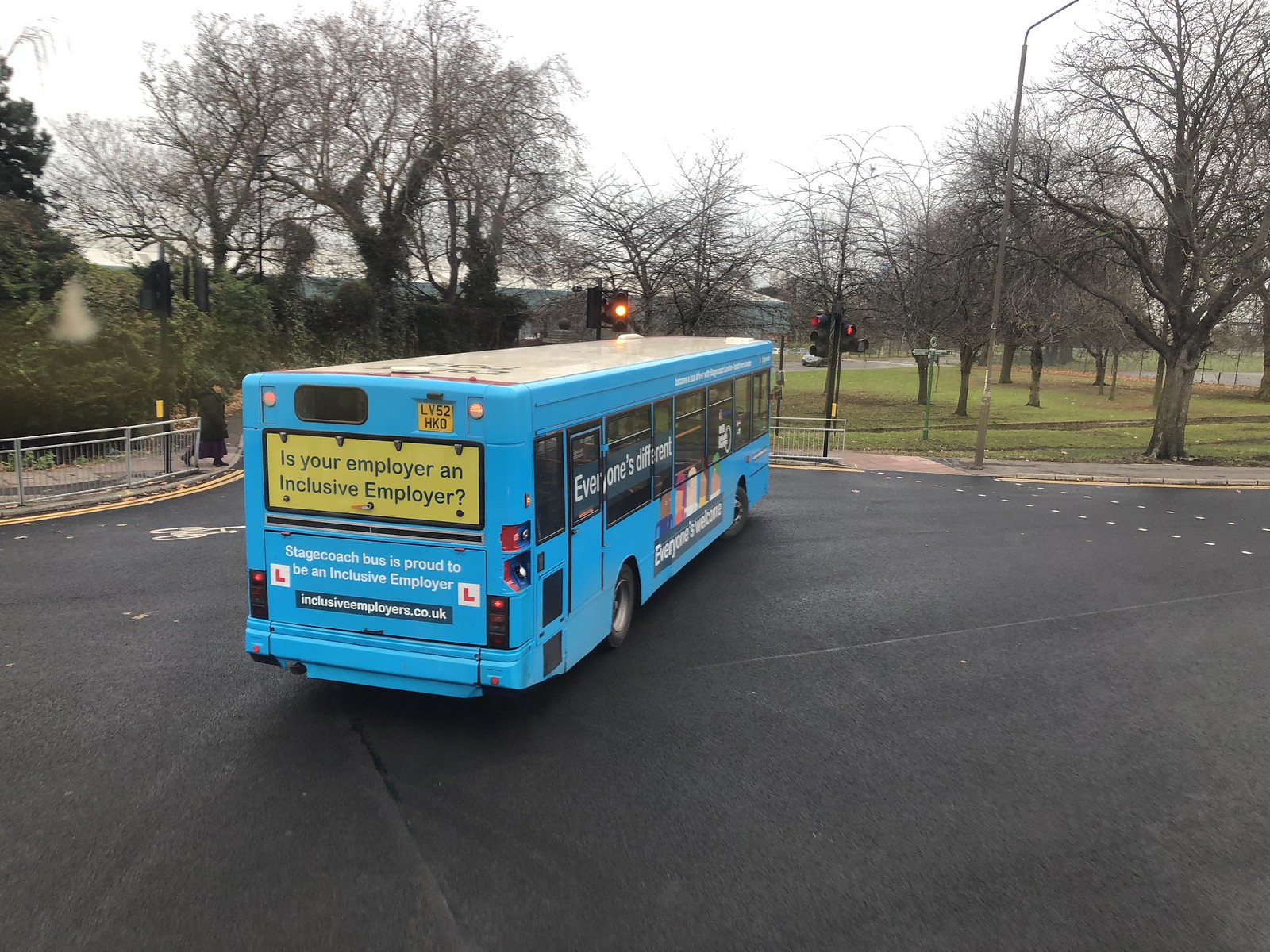This image depicts a vibrant, light blue Stagecoach bus with a white roof, captured from the rear. The bus is positioned in a large, black parking lot or a similar area, indicative of it being either stopped or parked. The backdrop features a gray sky typical of winter, given the leafless trees, along with some green grass. Nearby traffic lights suggest proximity to an intersection.

On the rear of the bus, a prominent yellow box with black text reads, "Is your employer an inclusive employer?" Directly below, in white text, it states, "Stagecoach Bus is proud to be an inclusive employer," with a blue box containing the website "inclusiveemployers.co.uk" underneath. A yellow license plate marked "LV52 HKO" is also visible. On the side windows of the bus, the phrase "Everyone's different" is painted, reinforcing the inclusivity message. The combination of these elements, and the UK-based website, suggests the image was taken in the United Kingdom.